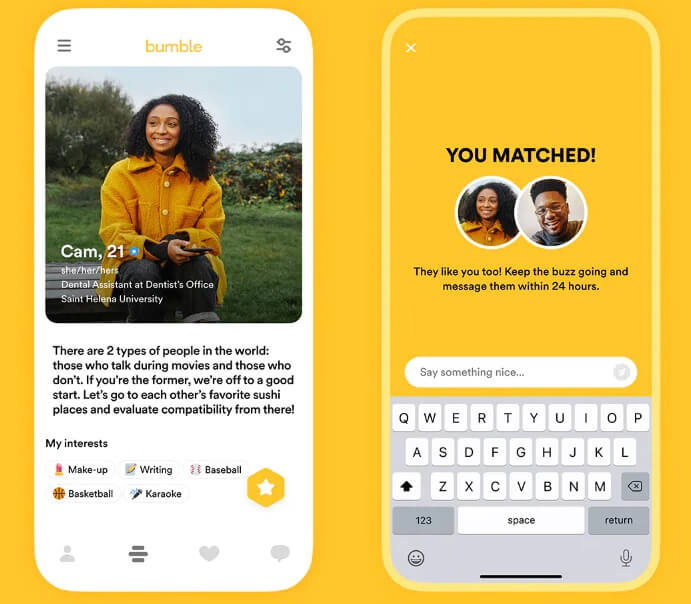In this detailed screenshot with a prominent yellow background, we observe a profile on a dating app, presumably Bumble. On the left side of the screenshot, there is an image of a young, dark-skinned female with curly black hair. She is wearing a yellow coat paired with rolled-up jeans and is seated on a bench, exuding a casual yet stylish look. Above her image, the word "bumble" is displayed in yellow text.

Overlaying her image are the following details: "Cam, 21, she/her/hers, dental assistant at dentist's office, St. Helena University." Below her image, there's a quirky personal message: "There are two types of people in the world: those who talk during movies and those who don't. If you're the former, we're off to a good start. Let's go to each other's favorite sushi places and evaluate compatibility from there."

On the right side of the screenshot, there's another image showcasing a match between Cam and a male individual. Their two faces are juxtaposed. Above their combined image, it reads "You matched" in black text. Below this, there is an encouraging note: "They like you too. Keep the buzz going and message them within 24 hours."

This detailed caption skillfully captures the essence of the dating interaction and the specific profile features in the app's user interface.